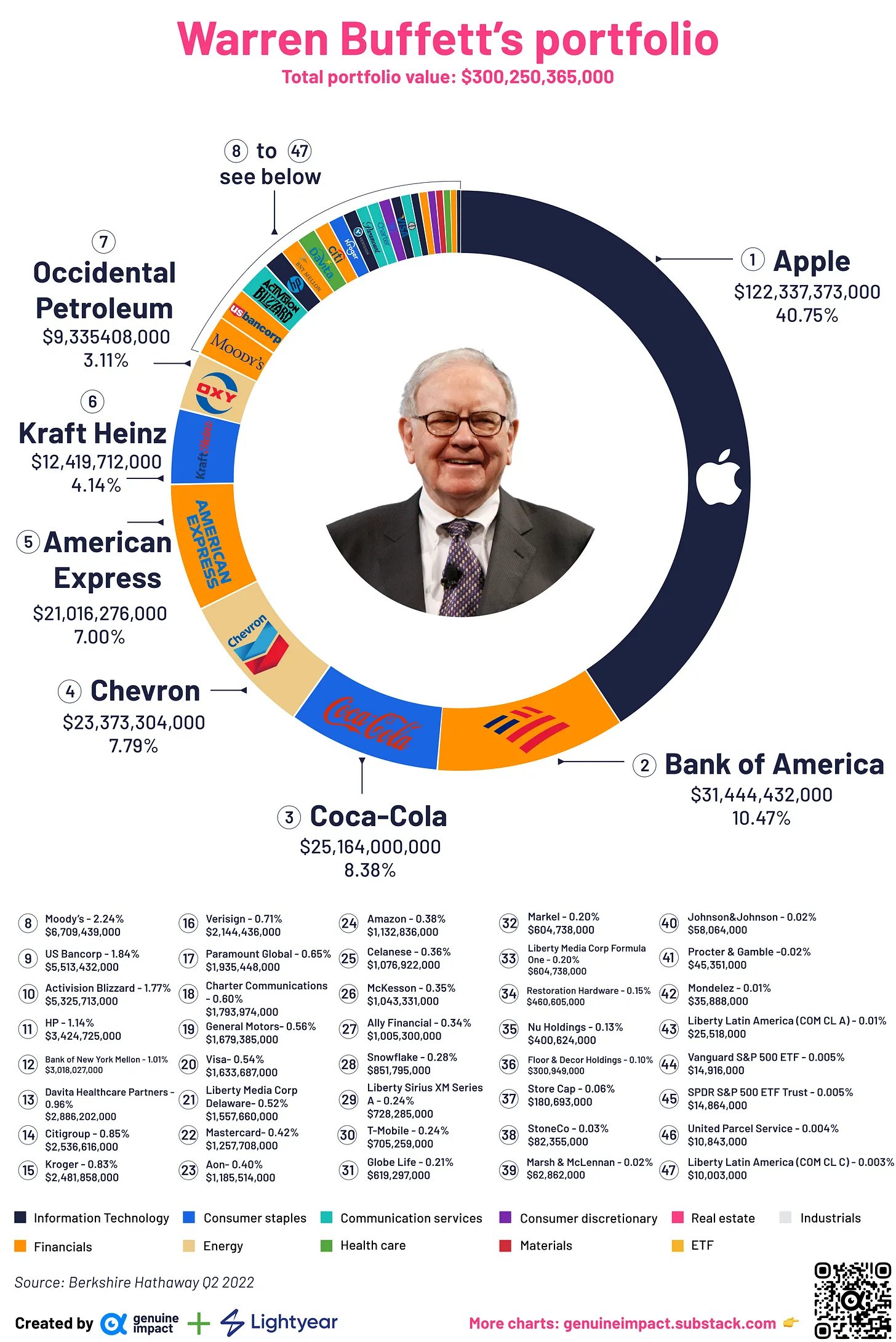This detailed diagram provides a comprehensive overview of Warren Buffett's portfolio. At the top, in pink lettering, it states "Warren Buffett's Portfolio" with a total portfolio value of $300,250,365,000. In the center of the diagram, there is an image of Warren Buffett himself, depicted as an older man with white hair, black glasses, and a gray suit paired with a paisley tie. Surrounding him is a large circular chart, color-coded to represent different segments of his portfolio.

The largest segment, occupying 40.75% of the circle, is Apple, valued at $122,337,373,000. Next is Bank of America, making up 10.47% of the portfolio, valued at $31,444,432,000. Following this is Coca-Cola, shown in light blue and red, comprising 8.35% of the portfolio at $25,225,164,000.

Other significant holdings include Chevron, American Express, Kraft Heinz, Occidental Petroleum, Moody's, U.S. Bancorp, and Activision Blizzard. These holdings gradually decrease in size and value, with smaller segments represented by companies like HP, Teva Healthcare Partners, Citigroup, Kroger, Verizon, Paramount Global, Charter Communications, and General Motors, among others. Beyond this point, each of the remaining companies constitutes less than 0.5% of the total portfolio.

At the bottom of the diagram, the source is credited as being created by Genuine Impact, with a mention of additional charts available on genuineimpact.substack.com.